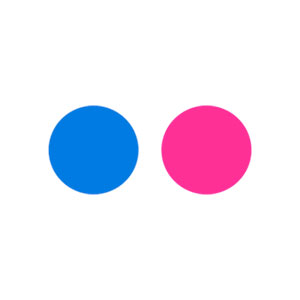This image features a completely white background with no border lines or text. Positioned centrally within the frame are two vivid circles, arranged side by side horizontally. On the left, there is a light blue circle, while on the right, a magenta circle sits adjacent to it. Both circles are of substantial size, contrasting sharply against the stark white backdrop. The simplicity of the design suggests that these colored circles may be part of a color utility or selection tool.